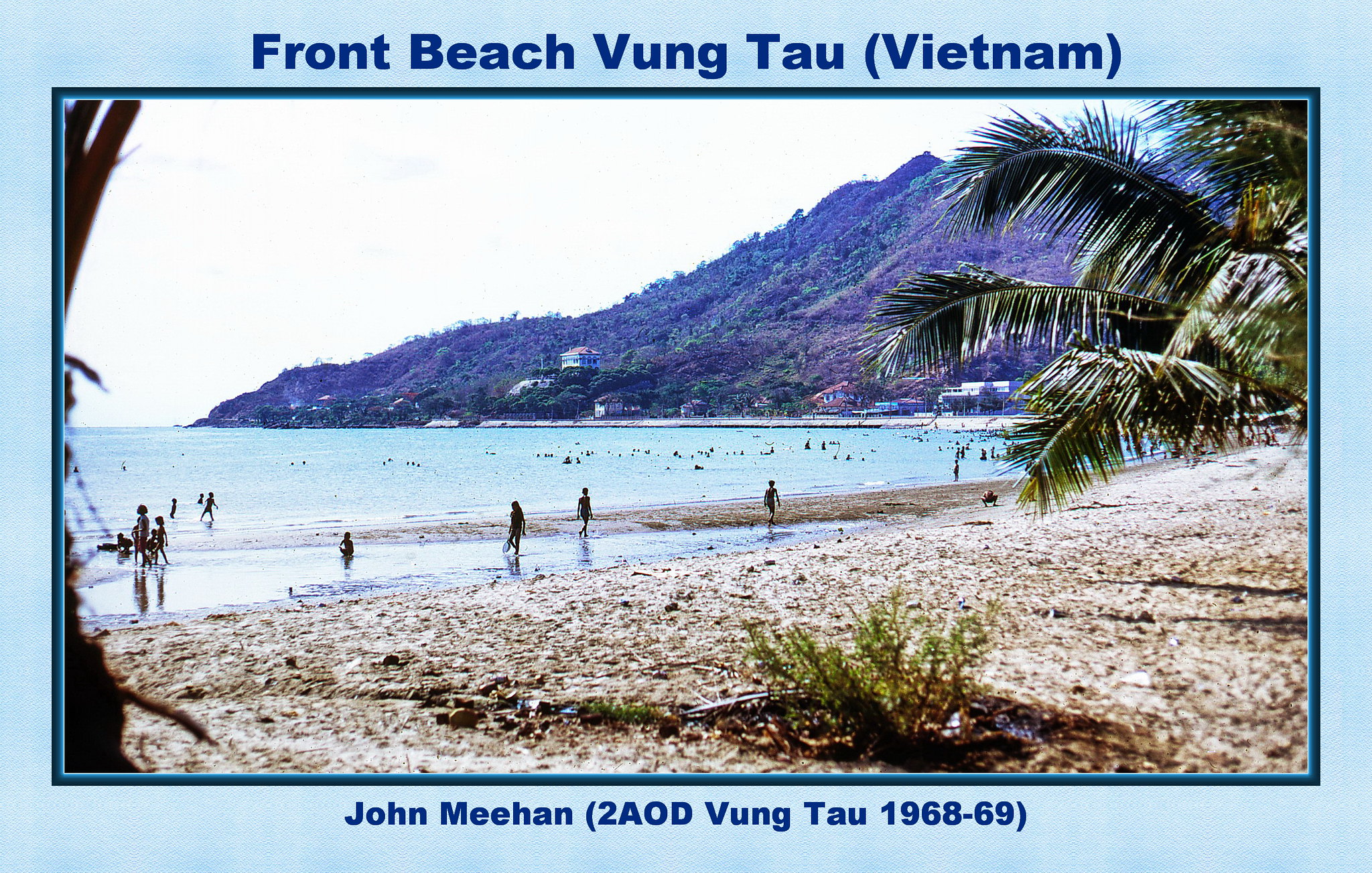The image resembles a vintage postcard, framed by a light blue border adorned with dark blue text. The top section of the border reads "Front Beach, Vung Tau (Vietnam)." Below the picture, the text "John Meehan (2AOD, Vung Tau, 1968-69)" is inscribed. The central photograph showcases a tropical beach scene. The foreground features sandy shores dotted with green shrubs and palm leaves extending from the upper right corner. In the middle left, there is the ocean, animated with numerous people walking along the shore and swimming in the water. The background reveals a sprawling shoreline with buildings and hills, wrapping around a large bay. Scattered black silhouettes in the water suggest more people swimming or floating. The overall composition evokes a serene yet lively coastal environment framed perfectly to capture a moment in time.